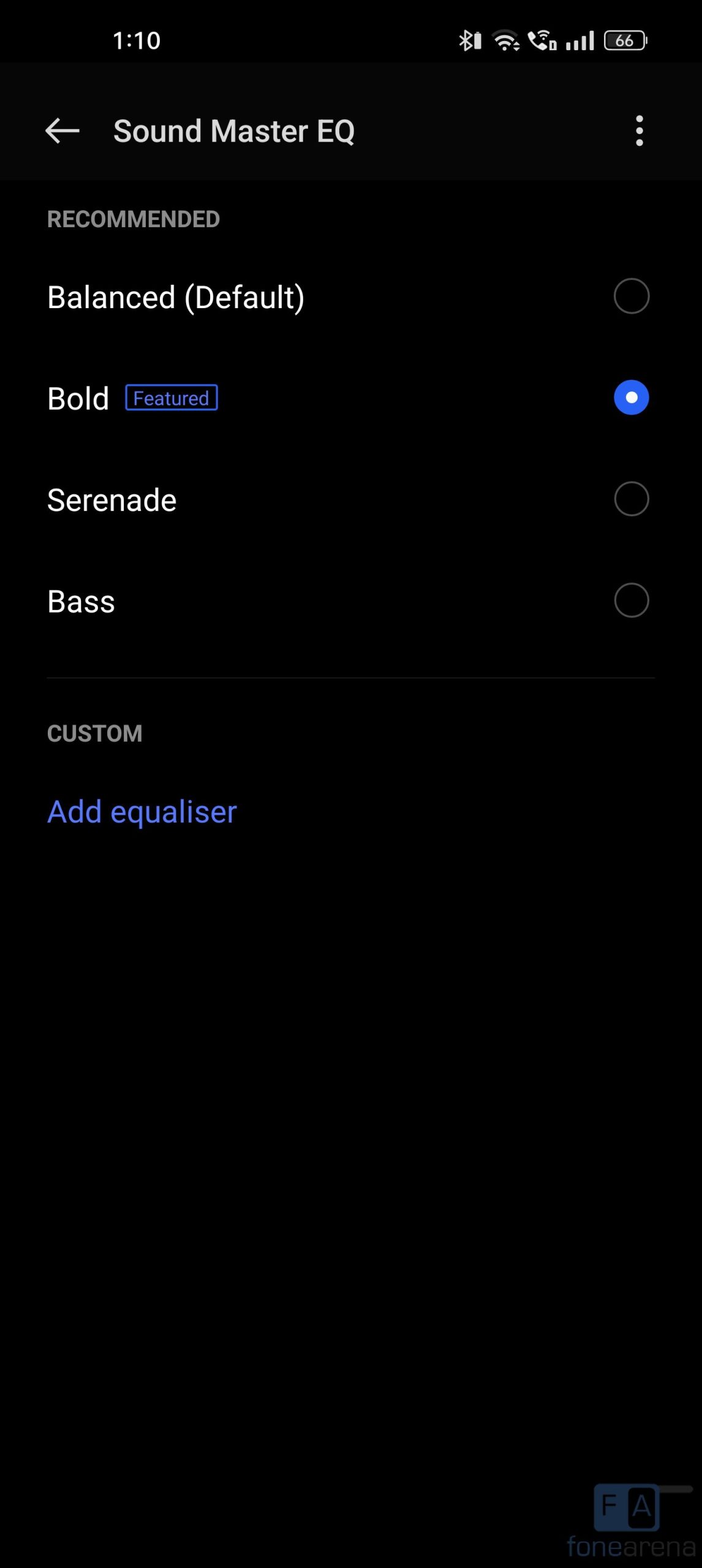In this detailed screenshot, the interface appears to be from a mobile device, set against a solid black background with white text. Located in the upper-left corner, the time is displayed as 1:10. Moving to the right, a series of icons can be seen in the following order: a Bluetooth icon, a Wi-Fi symbol indicating an active connection, a battery icon showing a full charge, and a signal strength meter with four bars indicating full reception.

Directly beneath these icons, the heading "Sound Master EQ" is prominently displayed. An arrow pointing to the left is positioned to the left of this heading, suggesting a navigation option. Below this, the smaller text reads "Recommended," followed by "Balanced Default" which is prominently shown as the current selection.

Further down, the word "Bold" is present and labeled as "Featured" within a blue box, signifying its importance or recommendation. To the right of this, a small circle is highlighted, indicating it is currently selected. Underneath, the options continue with "Serenade" and then "Bass." In a gray font on the left beneath "Bass," the word "Custom" is displayed. Directly below "Custom," in blue text, the option "Add Equalizer" is offered, providing users the ability to personalize their audio settings further.